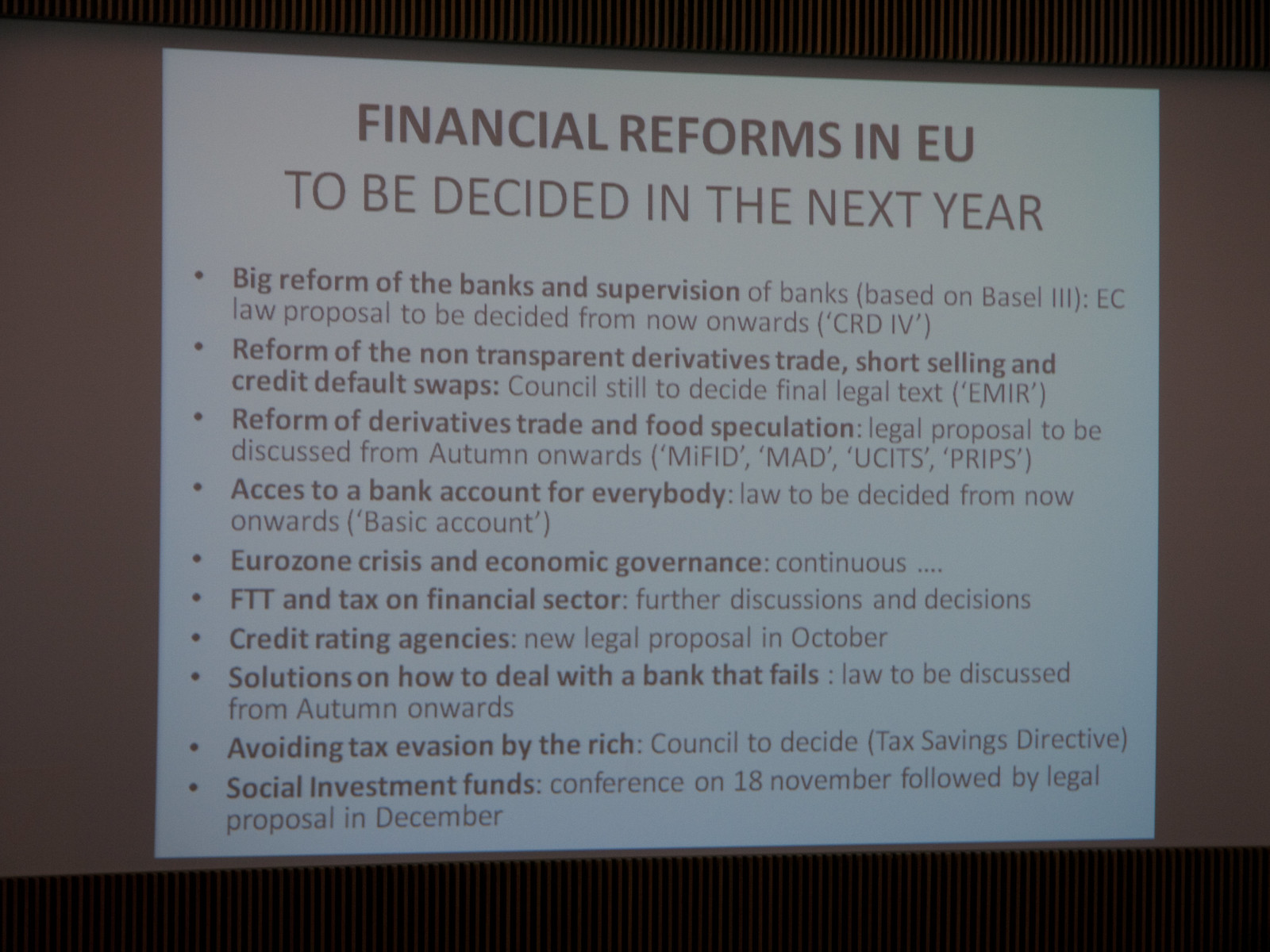The image depicts a PowerPoint presentation projected onto a screen, framed by black vertical bands. The central white rectangle displays dark, predominantly black text. At the top, the bold heading reads "Financial Reforms in EU." Below this, in lighter text, it states "to be decided in the next year." The presentation lists a series of extensive bullet points addressing upcoming financial reforms. 

1. **Big reform of the banks and supervision of banks:** Plan based on Basel 3 with legislative proposals to be decided from now onwards (referred to as CRD IV).
   
2. **Reform of non-transparent derivatives trade, short selling, and credit default swaps:** Final legal text, EMIR, subject to council decision.

3. **Reform of derivatives trade and food speculation:** New proposals to be discussed from autumn onwards.

4. **Access to bank accounts for everybody:** Legislative discussions are imminent.

5. **Eurozone crisis and economic governance:** Continuous discussions, including the Financial Transaction Tax (FTT) and broader taxes on the financial sector.

6. **Credit rating agencies:** A new legal proposal expected in October.

7. **Solutions for dealing with failing banks:** Law to be debated starting in autumn.

8. **Avoiding tax evasion by the rich:** Decision pending from the council.

9. **Social investment funds:** A conference scheduled on 18 November to be followed by a legal proposal in December. 

This presentation outlines significant upcoming financial legislative changes within the EU, highlighting a structured timeline for decisions and reforms spanning various financial sectors.